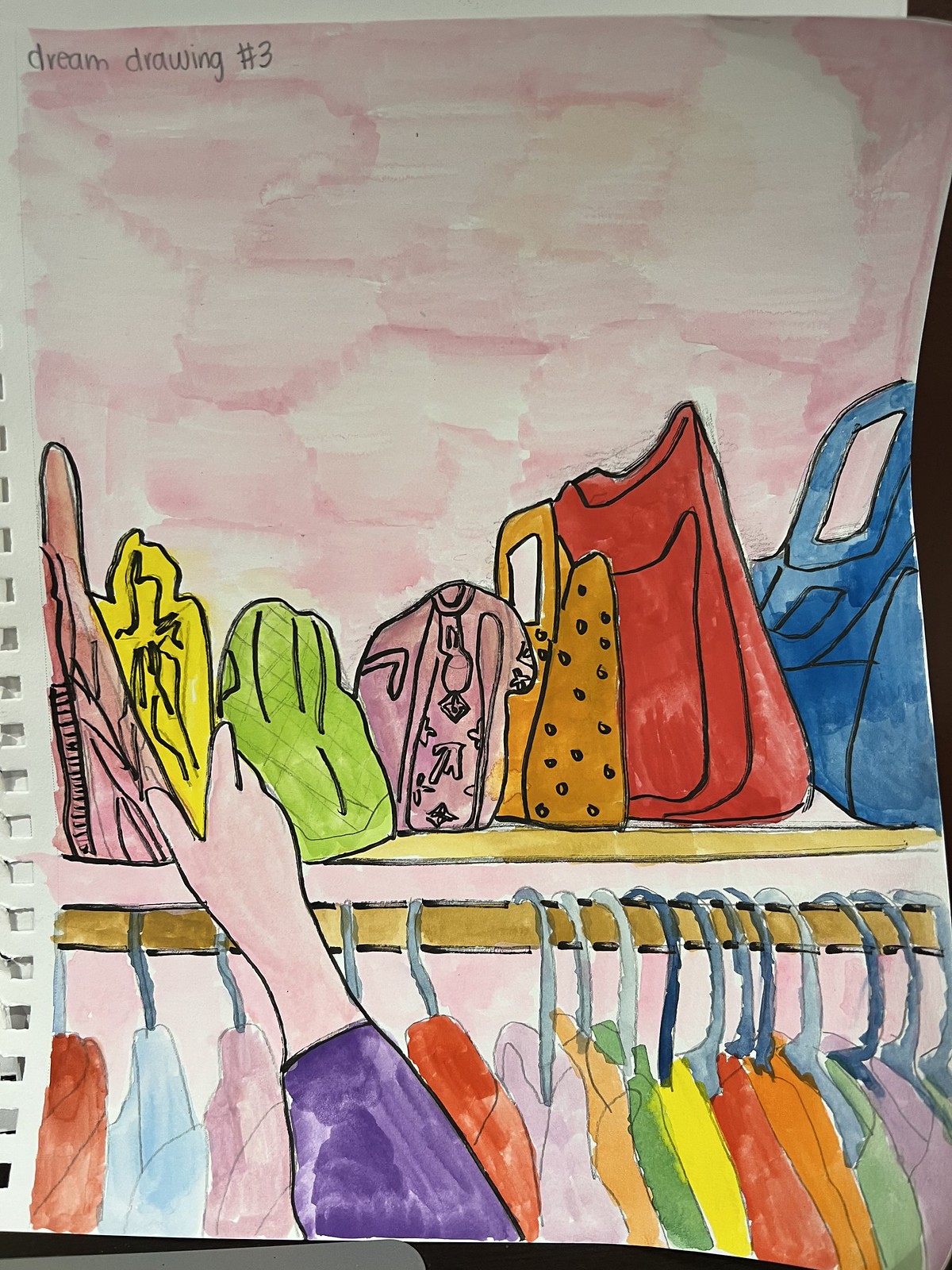The image showcases a detailed multimedia art piece created on a spiral notebook, evident from the rectangular holes on the left edge. The artwork is a color drawing outlined in magic marker and enriched with watercolor. At the top of the piece, in lowercase letters, the text "dream drawing number 3" is inscribed. A wash of varying shades of pink, resembling clouds, forms the background, implying the interior of a closet. 

Inside the closet, a shelf holds an array of multicolored handbags—purple, yellow, green, pink, orange, red, and blue—neatly aligned side by side. One yellow handbag stands out as a white-skinned hand in a loose purple sleeve reaches towards it. Below the shelf, a wooden pole extends horizontally, adorned with an assortment of clothing in diverse colors including red, blue, purple, brown, green, and yellow. These garments hang from silver hangers, their details simplified, only revealing the tops of the shirts. The composition vividly blends the dreamy, ethereal quality of the pink watercolor backdrop with the organized array of vibrant bags and clothing.